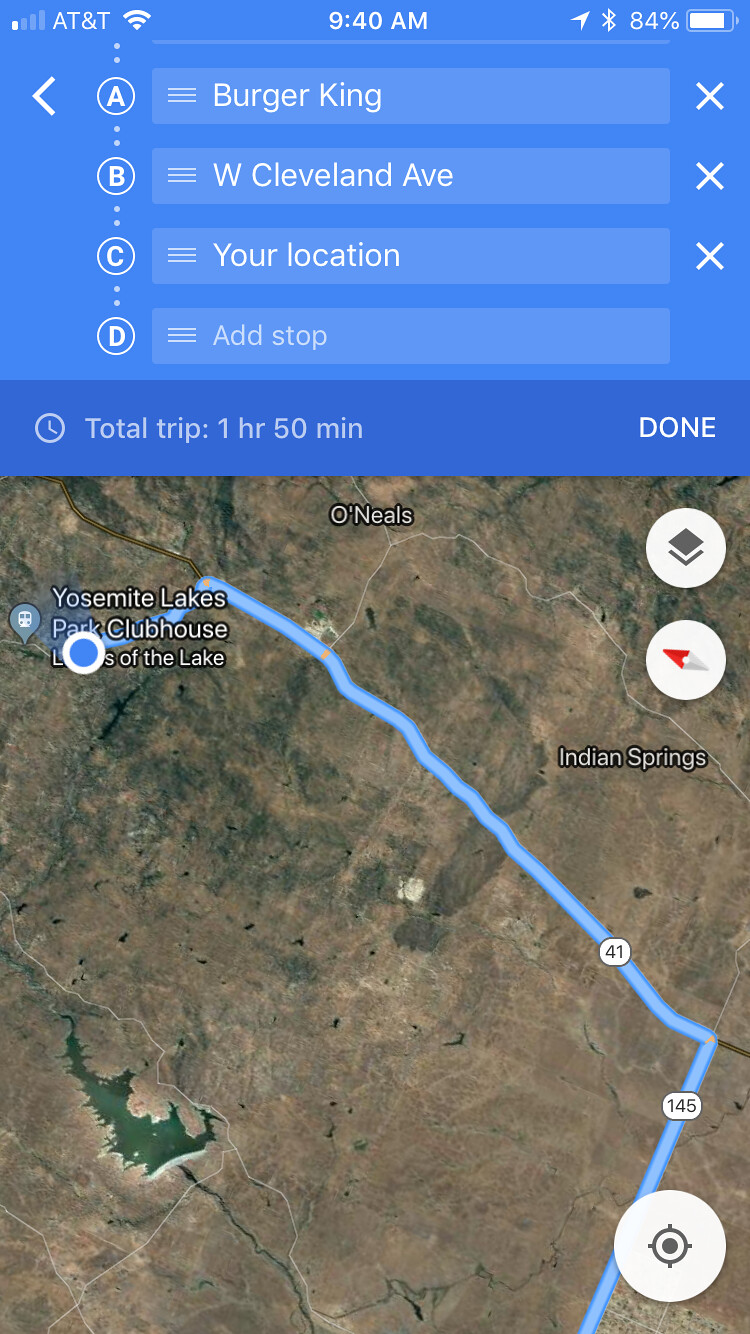This image is a detailed screenshot of a smartphone navigating a route in its Maps app. The phone, an AT&T device, shows connectivity to Wi-Fi with a single bar of service, and indicates it is 9:40 a.m. The status bar reveals that location services, Bluetooth, and Do Not Disturb mode are active, and the battery is at 84%. The Maps app is plotting a trip comprising multiple points: Point A is Burger King, Point B is West Cleveland Avenue, Point C is labeled "your location," and Point D is open for an additional stop. These details are within a blue box at the top of the screen, with the total trip duration listed as 1 hour and 50 minutes accompanied by the word "Done" next to a small clock icon. Below this, there is a detailed aerial map showing the initial point at Yosemite Lakes Park Clubhouse, highlighted with an icon. The map route, marked in blue, travels along Interstate 41 before switching to Route 145. Additional landmarks like Indian Springs and O'Neill's are visible to the north, with the map's color palette displaying brown, dark green, and light green hues to reflect terrain textures.